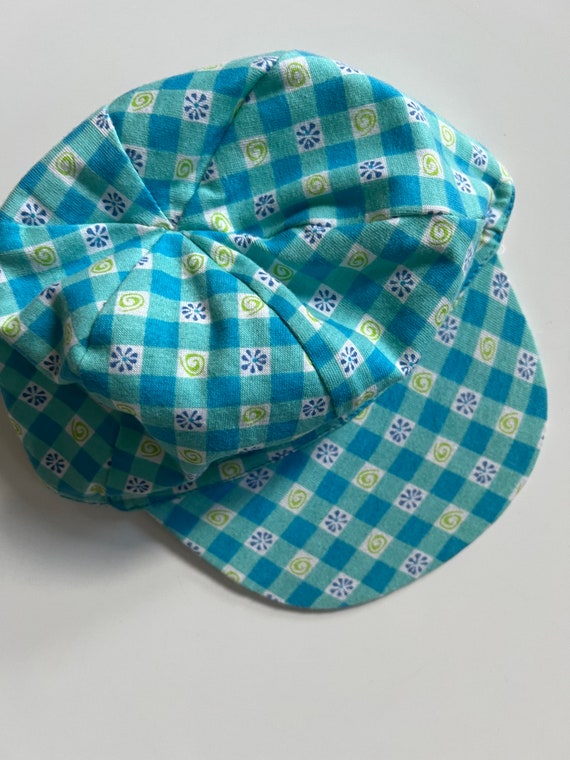The photograph captures a unique and detailed hat resting on a light gray or off-white surface. The hat features a checkered pattern composed of alternating light blue, dark blue, and white squares. Within the white squares, there are intricate designs: some depict lime green swirls, while others display formations of blue teardrops arranged in circular patterns, creating a floral or burst-like effect. The hat closely resembles a baseball cap due to its stiff bill, but its overall shape and soft, sunken cotton top suggest it may be a summer sun hat, perhaps something reminiscent of 1980s or 90s fashion. The detailed and vibrant patterns, including elements likened to hand-sewn flowers or bursts, add a distinct and nostalgic charm, making it a truly unique accessory.